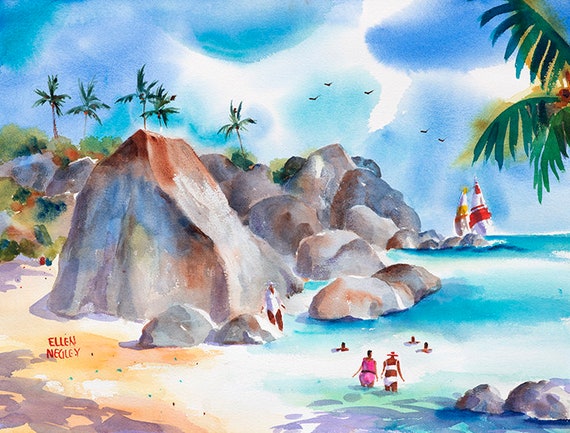This watercolor painting by Ellen Negley depicts a whimsically stylized, cartoonish beach scene viewed from an elevated perspective. The sky, adorned with light clouds, stretches over a vivid shoreline. Two colorful sailboats with striped sails—yellow and white, red and white—dot the horizon. The azure sea, tinged with white accents, laps up against the rocky beach marked by large boulders. In the foreground, two women wade thigh-high in the water, one in a pink bikini and the other in a white bikini with a hat. Nearby, another woman in a white one-piece bathing suit stands by the rocks, gazing toward the viewer. Additional swimmers frolic in the gentle waves while five birds soar in the sky overhead. Palm trees punctuate the skyline, contributing to the warm, soft, pastel hues that evoke a quintessential beach atmosphere. Despite its rich detail, the scene's vibrant colors and exaggerated forms firmly place it in the realm of expressive, stylized art rather than a realistic portrayal.